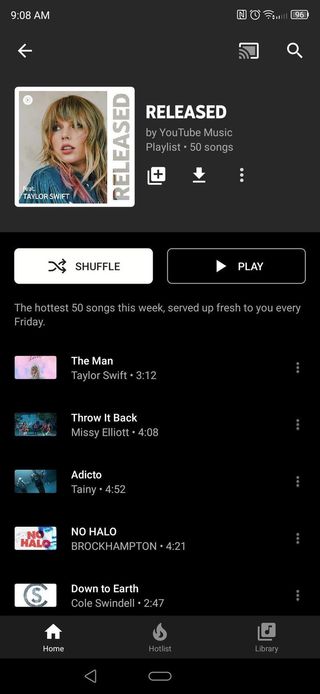This image is a screenshot from a phone displaying the YouTube Music app. The screen showcases a playlist named "Released," which features a total of 50 songs. The topmost entry in this playlist is a song by Taylor Swift, prominently highlighted with an album cover image of her in a square icon next to the playlist title "Released."

In the midsection of the screen, there is an indication that the user has engaged the "Shuffle" function, which is highlighted in white, contrasting against the black "Play" button that features a right-pointing arrow.

Further down, the screen displays the playlist description, stating it includes "The hottest 50 songs this week," and mentions that this selection is "served up fresh to you every Friday." Each song listed has a thumbnail image of its respective music video, followed by details including the song title, artist, and duration. To the far right of each song entry, there is a vertical ellipsis (three dots) menu for additional options.

Among the song titles listed, there are "The Man," "Throw It Back," "A Dicto," "No Halo," and "Down to Earth."